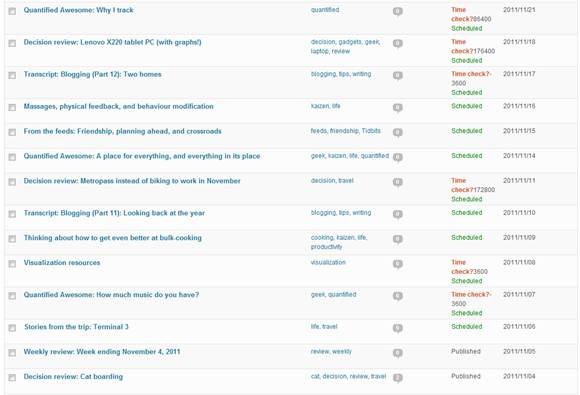The website features a predominantly whitish-gray background and is organized into several rectangular columns of text. On the far left, there is a series of blue text boxes starting from the top with titles that read "Quantified Awesome," "Why I Track," "Decision Review," "Lenovo X220 Tablet PC with Graphics," followed by "Transcript Blogging Part 12: Two Homes," and lastly, "Massages: Physical Feedback and Behavior Modification." 

In the center of the page, additional blue text boxes are present. Moving to the right, various text in red and green hues can be seen, providing additional context or highlighting different sections. On the far right, gray-colored text appears to display dates and other relevant information.

Each of these text columns is accompanied by a gray square to their left side, which resembles a checkmark box that could presumably be marked off.

Despite having observed the page for about 90 seconds, the exact purpose of this website remains unclear.